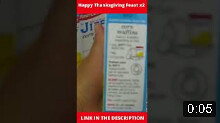This small, predominantly brown image appears to depict an information board situated in a public space. The board is mounted on a post topped with a square structure. A red header with white, illegible text adorns the top of the sign, while a matching red stripe with similarly unreadable white text runs along the bottom. The image is angled to reveal two sides of the board: the left side features a map accompanied by minuscule writing; the right side is densely packed with text enclosed within a blue border. Notably, the corner of the text section is marked with the number "005."